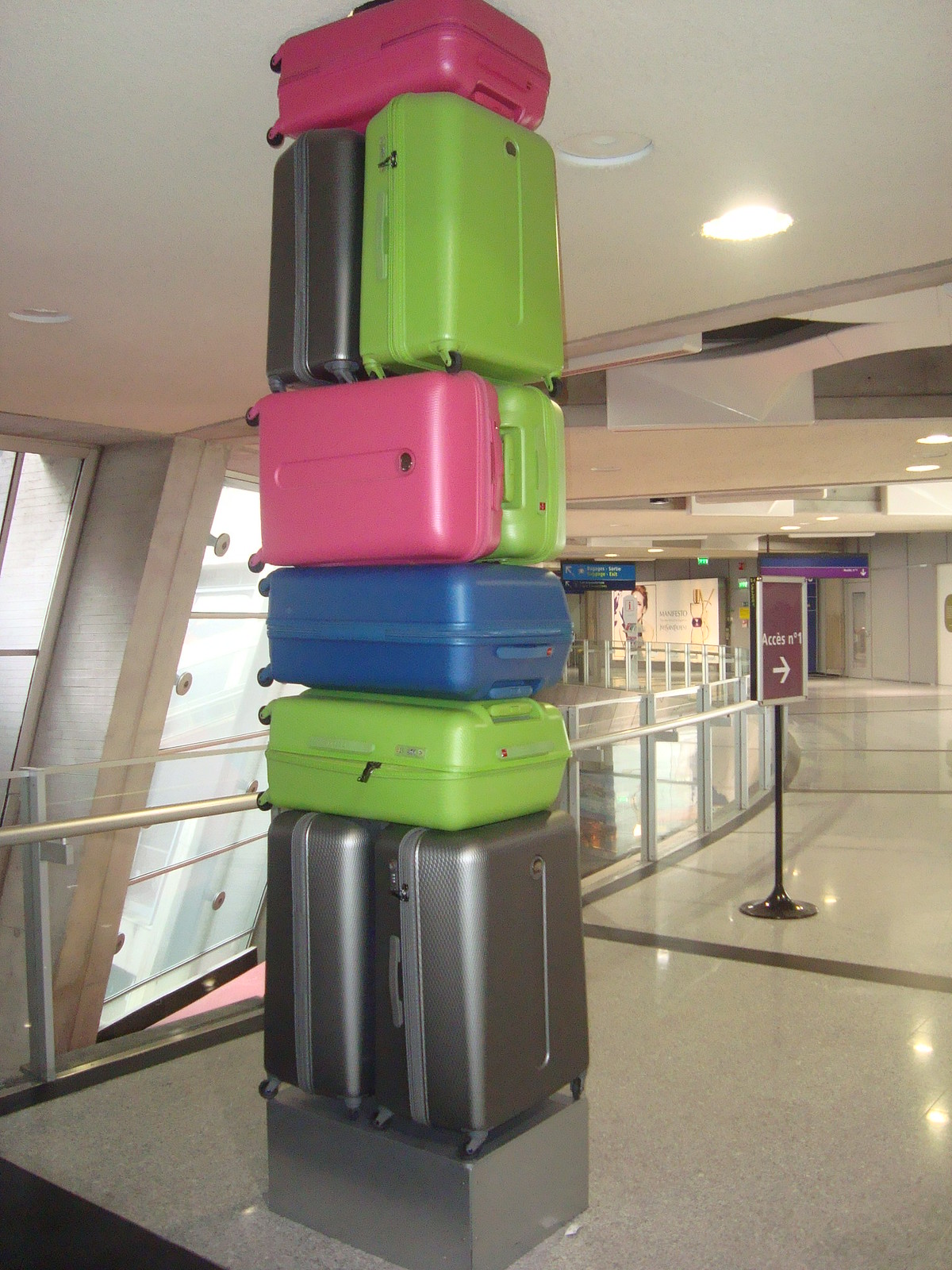The image depicts a strikingly tall stack of hard-shell suitcases, meticulously arranged in the hallway of an airport. The suitcases are stacked on a small gray pedestal with a shiny, polished floor beneath them. At the base of the stack are two gray carry-on suitcases positioned side by side, standing vertically. Atop these, a vibrant green suitcase is laid horizontally, followed by a blue suitcase. Above the blue suitcase, a lime green and a hot pink suitcase lie side by side. Further up, a blue and a lime green suitcase are placed vertically. Capping the stack is a bright pink suitcase positioned horizontally.

The background reveals an airport corridor characterized by a glass and metal railing lining the walkway. A sign with a white arrow pointing forward and the word "access" is visible, along with a small figure in the far distance. This scene captures an unusual yet organized display of multicolored luggage against the sleek backdrop of an airport setting.